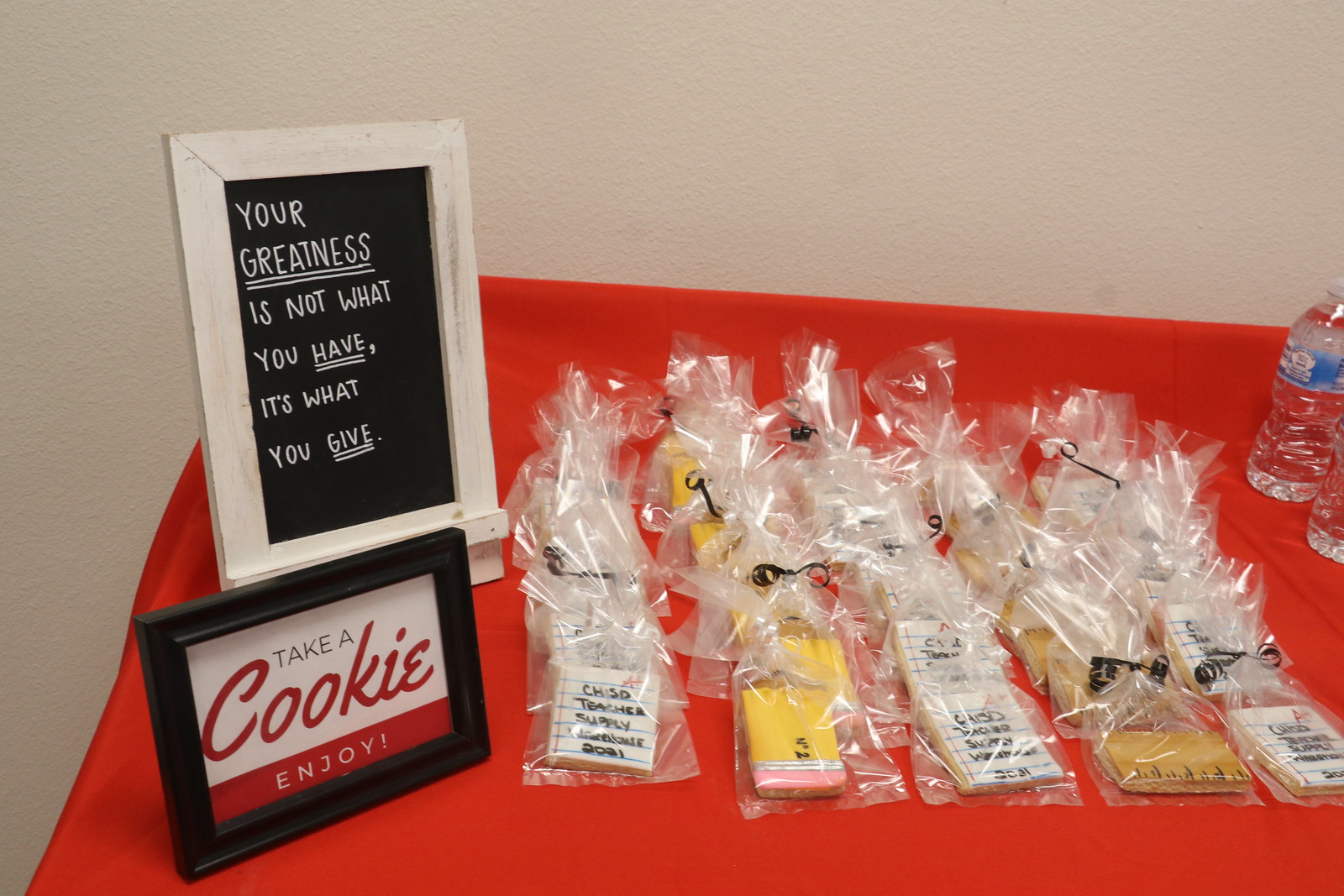The detailed image features an indoor scene showcasing a table adorned with a vivid red tablecloth against an off-white, beige wall with an orange peel texture. The centerpiece of the table consists of several individually wrapped items in cellophane bags tied with black ribbons, resembling cookies decorated to mimic pieces of paper, pencils, and rulers. On the right side of the table, two water bottles are prominently displayed. On the left side, there are two framed signs: the one in the back features a white frame with a mini chalkboard inscription that reads, "Your greatness is not what you have, it's what you give," while the smaller, black frame in the front bears the message, "Take a cookie," in black and red text, followed by "enjoy" in white text on a red background. The image offers a clear, detailed depiction of a thoughtfully arranged display table, emphasizing its colorful and purposeful decor.